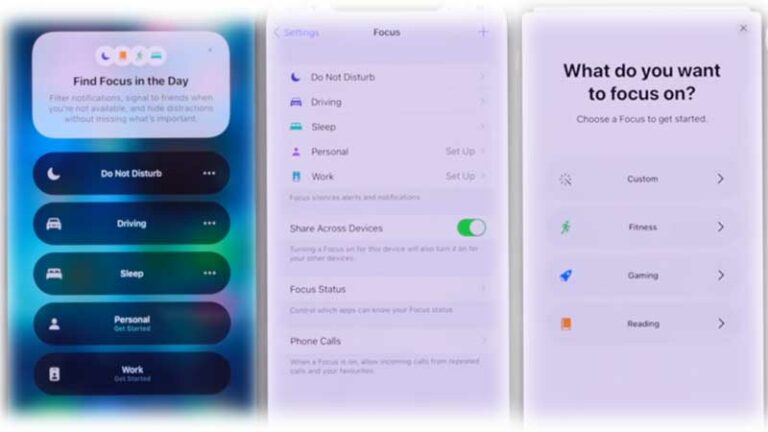This image series showcases various settings within an Apple device, most likely an iPhone, focusing on privacy and focus configurations.

**First Image: Overview of Focus Settings**
The initial image presents the main Focus settings interface, featuring multiple options such as "Do Not Disturb," "Driving," "Sleep," "Personal," and "Work." Additionally, there is a search bar available for users to delve deeper into each specific focus mode setting.

**Second Image: Detailed Focus Settings**
The second image provides a closer look at the Focus settings. Here, the user has selected to explore the Focus settings in detail, revealing the same options— "Do Not Disturb," "Driving," "Sleep," "Personal," and "Work." Users can toggle these functions on or off from this screen.

**Third Image: Customizing Focus Preferences**
The third image dives even deeper into the Focus setting customization. The screen prompts the user with the question, “What do you want to focus on?” and presents various customizable options like "Fitness," "Gaming," and "Reading." Users can presumably set goals or specific parameters for each focus area, tailoring their device to support their chosen activities and priorities.

Each image collectively provides a comprehensive view of how Apple devices allow users to manage their focus and privacy settings efficiently.